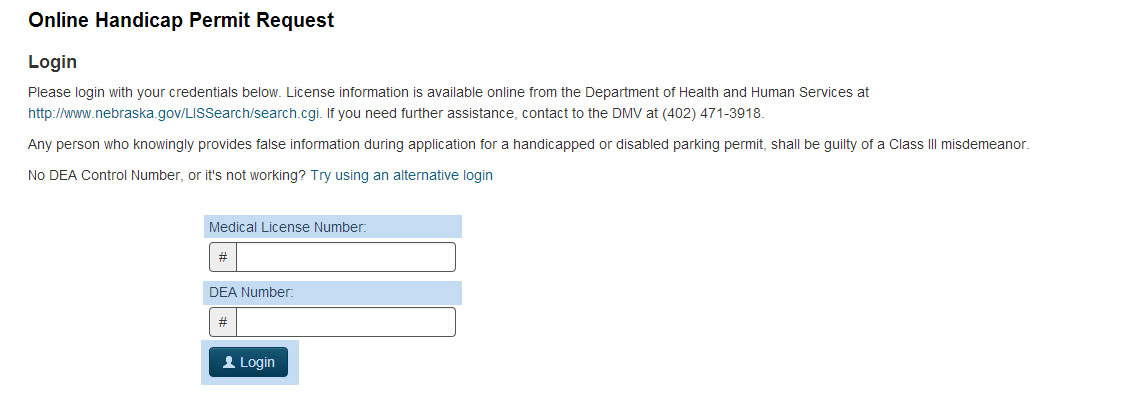The image shows a webpage prompting users to log in for an online handicap permit request. The message reads: "Please log in with your credentials below. License information is available online through the Department of Health and Human Services at http://www.nebraska.gov/U.S.search. For further assistance, please contact the appropriate department. Thank you."